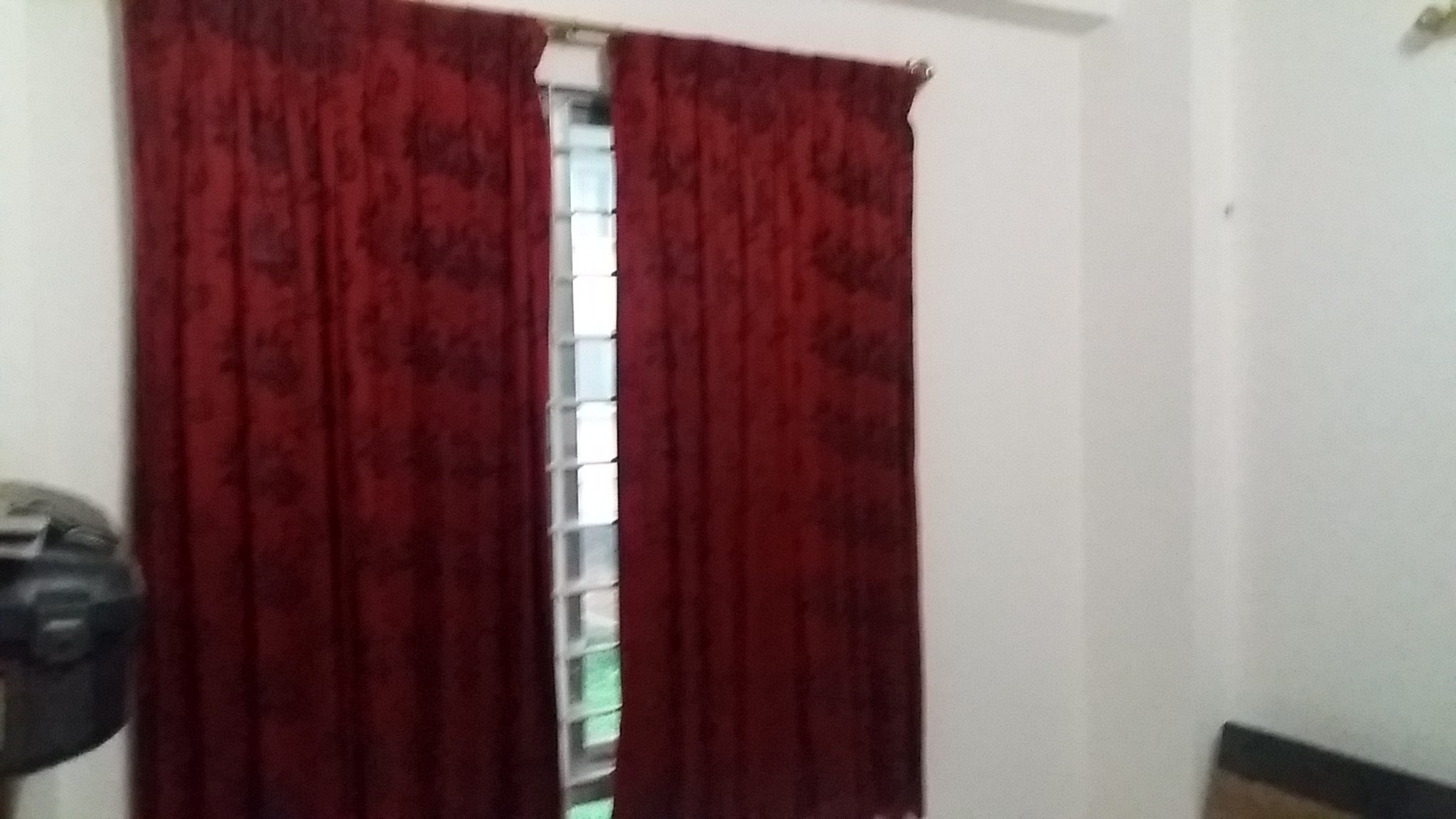The photograph captures the inside of a room with a whitish-gray wall featuring a window that is mostly obscured by a pair of long, deep red curtains with darker red flowery accents. The curtains, which are brick red to maroon in color, partially reveal a window equipped with open louvers or Venetian blind type shades. The image appears somewhat blurry, making it difficult to clearly identify certain elements. Through the window, a patch of green grass is visible, indicating that the room is likely on the first floor of the building. In the bottom right corner of the photograph, there is an indistinct object leaning against the wall, while to the left of the curtains, another black and potentially silver-colored object—which might be a printer or a paper shredder—can be seen, though it's not entirely identifiable due to the blurriness of the photo.